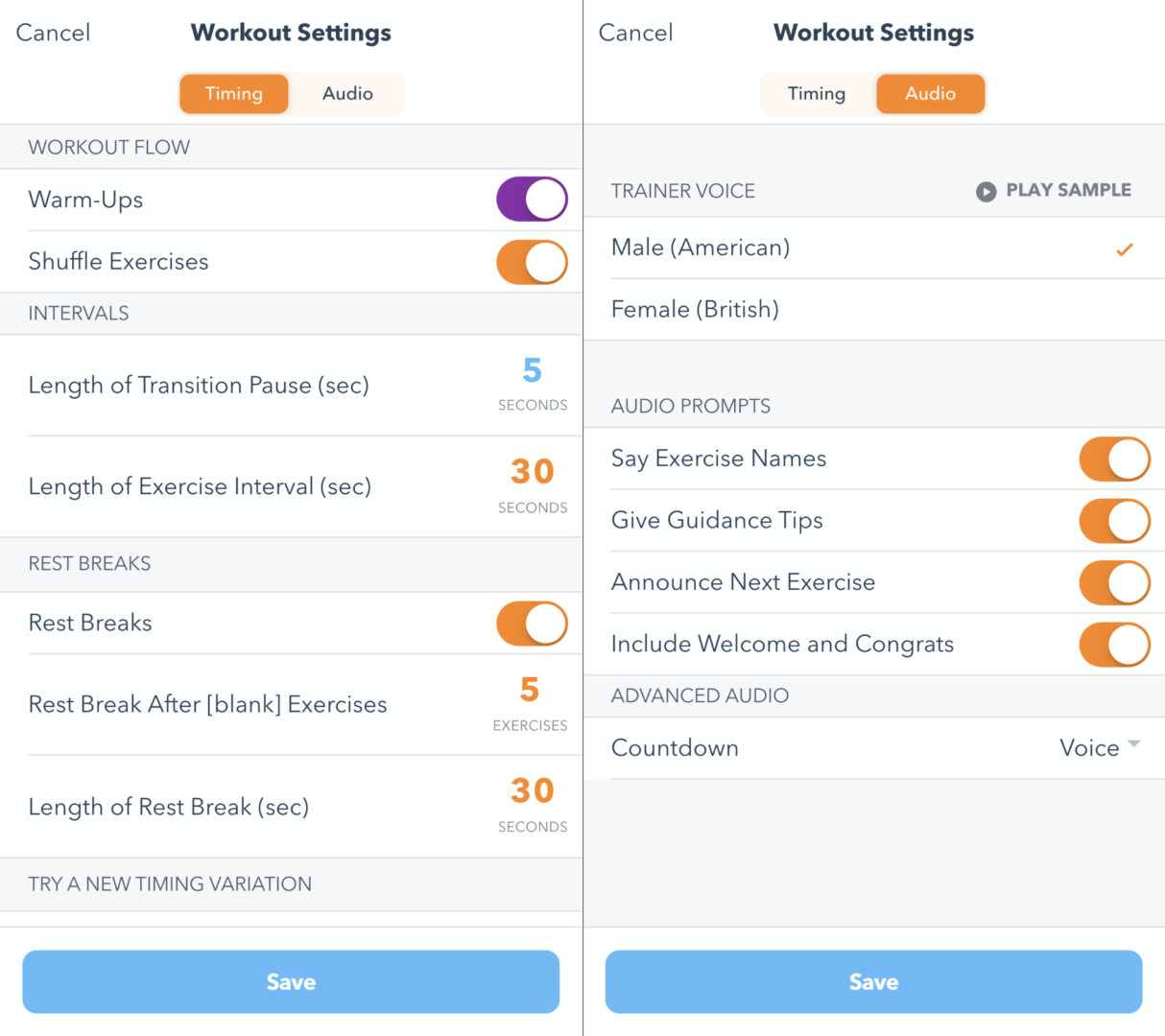Here is a detailed and cleaned-up caption for the image:

---

The image consists of two mobile phone screenshots placed side by side. We'll focus first on the screenshot on the left:

At the very top of the screen, in black font, there is the word "Cancel." Centered below, with bold black font, the header reads "Workout Settings" against a white background. 

Underneath the header, there are two selectable buttons labeled "Timing" and "Audio," with the "Timing" option selected. 

Below these buttons is a gray rectangular section titled "Workout Flow." Within this section are two white rectangular toggle options: "Warm-ups" (toggled on) and "Shuffle Exercises" (also toggled on). 

Another gray rectangle is present below labeled "Intervals," followed by a white rectangular section that specifies the "Length of Transition Pause (SEC)," set to "5 seconds." 

Further down, another white rectangular section indicates the "Length of Exercise Interval (SEC)," set to "30 seconds." 

Continuing downwards, a gray rectangle labeled "Rest Breaks" is followed by another white rectangular toggle option titled "Rest Breaks," which is toggled on. 

Next, there is a white rectangular section detailing the "Rest Break After __ Exercises" parameter, indicating "5 exercises." Below this, another white rectangular section specifies the "Length of Rest Break (SEC)," which is set to "30 seconds."

Towards the bottom of the screenshot, there is another gray rectangle labeled "Try a New Timing Variation," and below this is a prominent blue button labeled "Save."

---